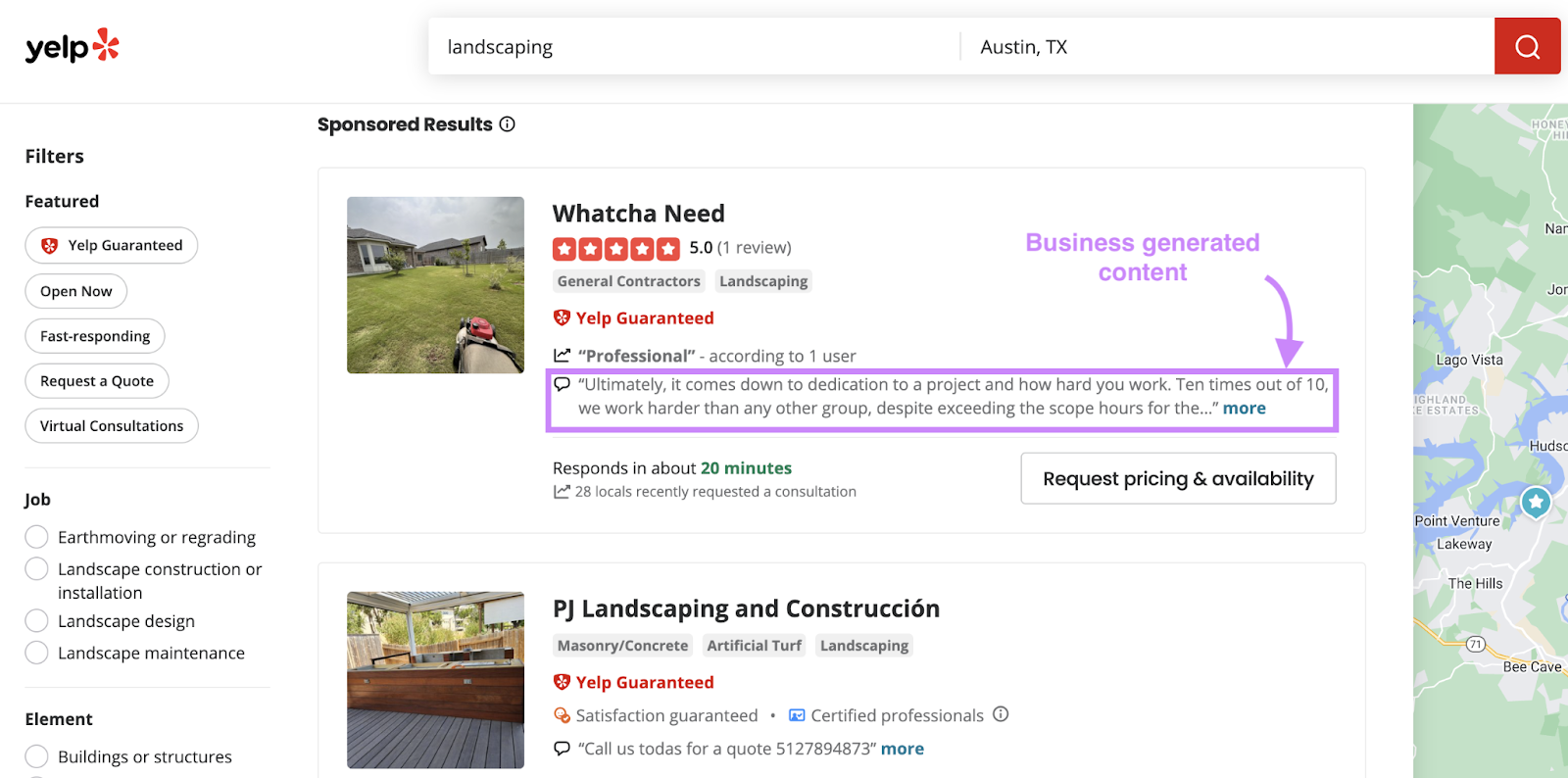This screenshot showcases a Yelp page featuring various businesses. Central to the image is a highlighted section outlined in purple. Above this rectangle, a purple arrow points downward to some text labeled "Business Generated Content." Inside the purple-highlighted area, there's a message from a business, though it is partially cut off: "Ultimately, it comes down to this decision to a project and how hard you work. Ten times out of ten, we work harder than any other group, despite exceeding the scope of hours." This appears to be a testimonial or statement emphasizing the business's commitment and work ethic.

The highlighted business is called Watch and Need, boasting a five-star rating with only one review. The service categories listed are General Contractors and Landscaping, and the business is marked as Yelp Guaranteed. According to one user review, they are regarded as professionals. The accompanying picture shows a residential yard with a lawnmower in operation.

Below this, the page features another business, PJ Landscaping and Construction. This business has an image showcasing a back deck with a hot tub, creating an inviting outdoor space. They are also identified as Yelp Guaranteed, Satisfaction Guaranteed, and Certified Professionals. Their description includes an invitation to call them for a quote.